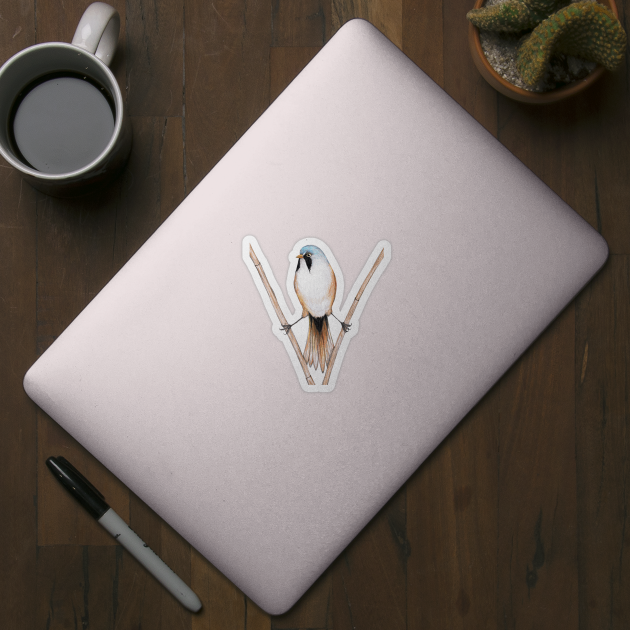The image is a high-resolution color photograph, viewed from above, capturing a neatly arranged scene on a dark wood tabletop. At the center of the composition is a closed silver laptop, positioned at an angle with its sides facing the bottom left and top right of the image. Prominently displayed in the middle of the laptop’s lid is a detailed sticker of a bird. The bird has a striking appearance with a blue head, white body, and brown feathers. Black stripes run beneath each eye, and it has a long, feathered tail that transitions from brown at the top to a lighter, grayish tone at the bottom. The bird is perched with one foot on each of two branches that form a V shape beneath it.

Surrounding the laptop, various items are strategically placed. To the top left is a white ceramic coffee mug, filled to the halfway mark with coffee, its handle oriented towards the top edge of the frame. The top right of the image features a small terracotta pot containing a dark green cactus. Adjacent to the bottom left corner of the laptop lies a black Sharpie pen, providing a touch of practicality to the scene. The overall aesthetic is minimal yet detailed, balancing elements of nature with technology against a rich, wooden background.